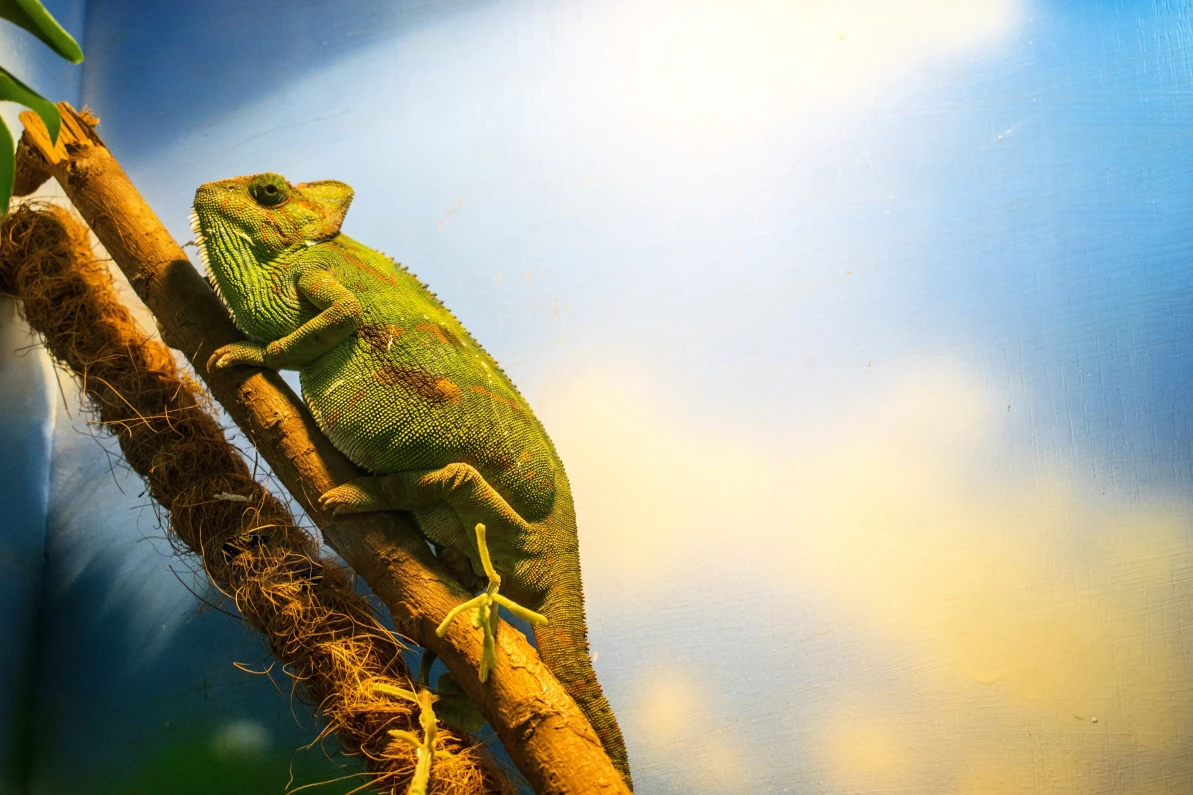The image showcases a vividly green iguana lying on a wooden branch, located on the left side of the picture. The branch, which has a mix of thin, leafy stems and a more substantial, traditional wooden branch on top, supports the iguana. The iguana itself has a slightly plump body with scattered orange and reddish-brown stripes. The background of the image is an artificial deep blue, with a bright white patch suggesting sunlight filtering through. The background features both shaded and bright blue areas, hinting at a digital or artistically altered origin. The scene is likely set within an enclosure, indicated by a visible divider in the corner, reinforcing the controlled environment.